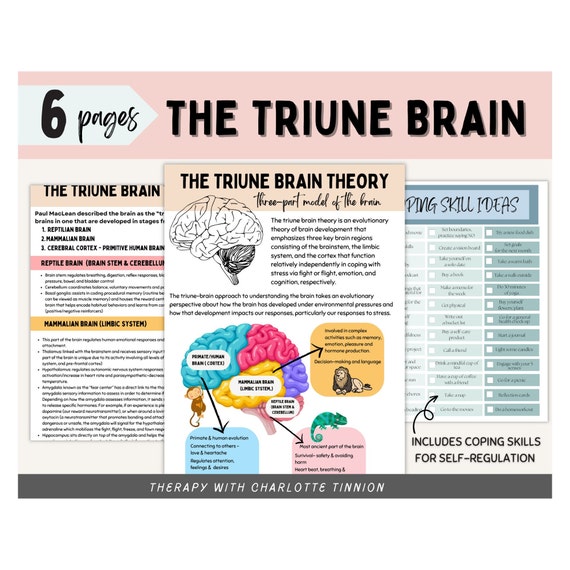The image is a detailed educational pamphlet cover, displayed in a rectangular horizontal frame. A pink banner spans the top, featuring the title "THE TRIUNE BRAIN" in uppercase black font. To the left of the banner, a small white block indicates "six pages" in black font. Centrally located beneath the banner is a vertical rectangle proclaiming "THE TRIUNE BRAIN THEORY: THREE-PART MODEL OF THE BRAIN," with "TRIUNE BRAIN THEORY" highlighted in bold uppercase and the rest in cursive font. Surrounding the central block, overlapping slightly, are additional pages that appear to be part of the pamphlet’s interior. These pages display various illustrations of the brain, including both black-and-white and colored models with arrows pointing to labels. Accompanying these illustrations is a small paragraph of text. The bottom of the graphic features a gray footer with white capital font reading "Therapy with Charlotte Tinian." The left side of the pink banner has a white arrow pointing left, reiterating "six pages" in black font. The overall layout includes informational content about Paul MacLean's Triune Brain Theory, illustrating the brain's development in stages: reptilian brain, mammalian brain, and cerebral cortex, with detailed charts and text explaining each section.